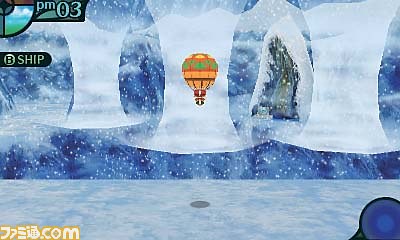The image is a pixelated screenshot from a retro-style video game, set in an icy, Arctic environment under a snowstorm or blizzard. Prominently, a yellow hot-air balloon accented with orange and green ascends in the center. Below, a tiny dot indicates its shadow on the ground. To the front of the balloon, three tall, white, tornado-like ice structures rise from glowing holes. The background features a frozen cave with stalactites and a blue interior. Little white dots throughout the image reflect the falling snow. In the top left corner, the text "PM 03" is visible, with “B ship” beneath it. The bottom left corner displays text, apparently in an Asian language, next to ".com" outlined in yellow. Lastly, a blue circle is in the bottom right-hand corner, contributing to the detailed game interface.